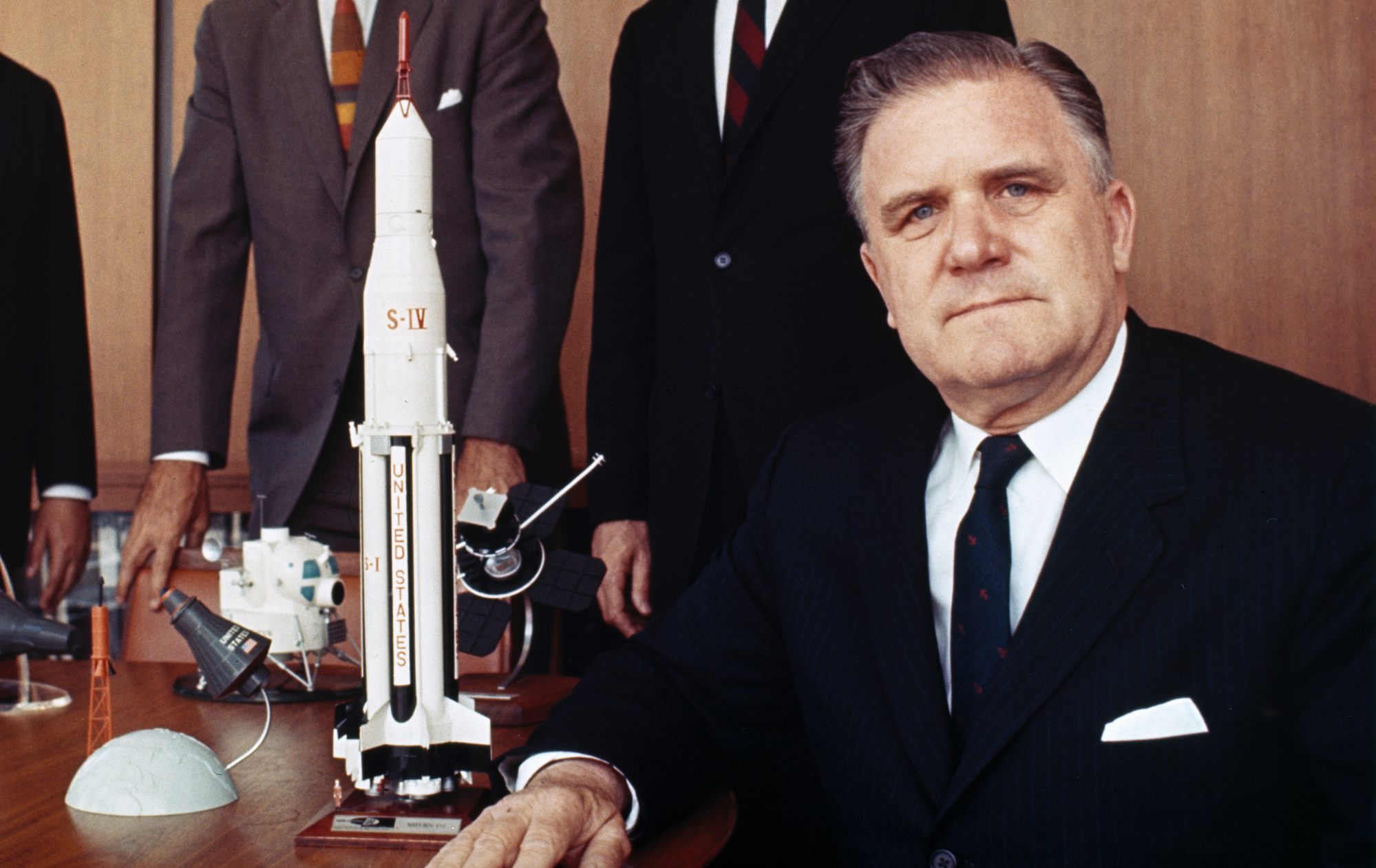This photograph captures what appears to be NASA scientist James Webb, after whom the renowned telescope is named, seated at a wooden table adorned with various models of spacecraft and satellites. Webb is distinguished by his dark blue suit, white dress shirt, white handkerchief in his breast pocket, and blue tie. His slicked-back, graying hair and blue eyes are prominently visible as he stares directly into the camera. His right arm rests on the table, drawing attention to the detailed spacecraft models, including a notably large white propulsion system marked with "SIV" or "S4" and "United States" in vertical red lettering. Behind Webb, three other men, blurred in the background, are seen wearing business suits—one in black, one in gray, and another in black—though only their torsos are visible. The scene underscores a scientific and collaborative environment, focusing on aerospace technology.